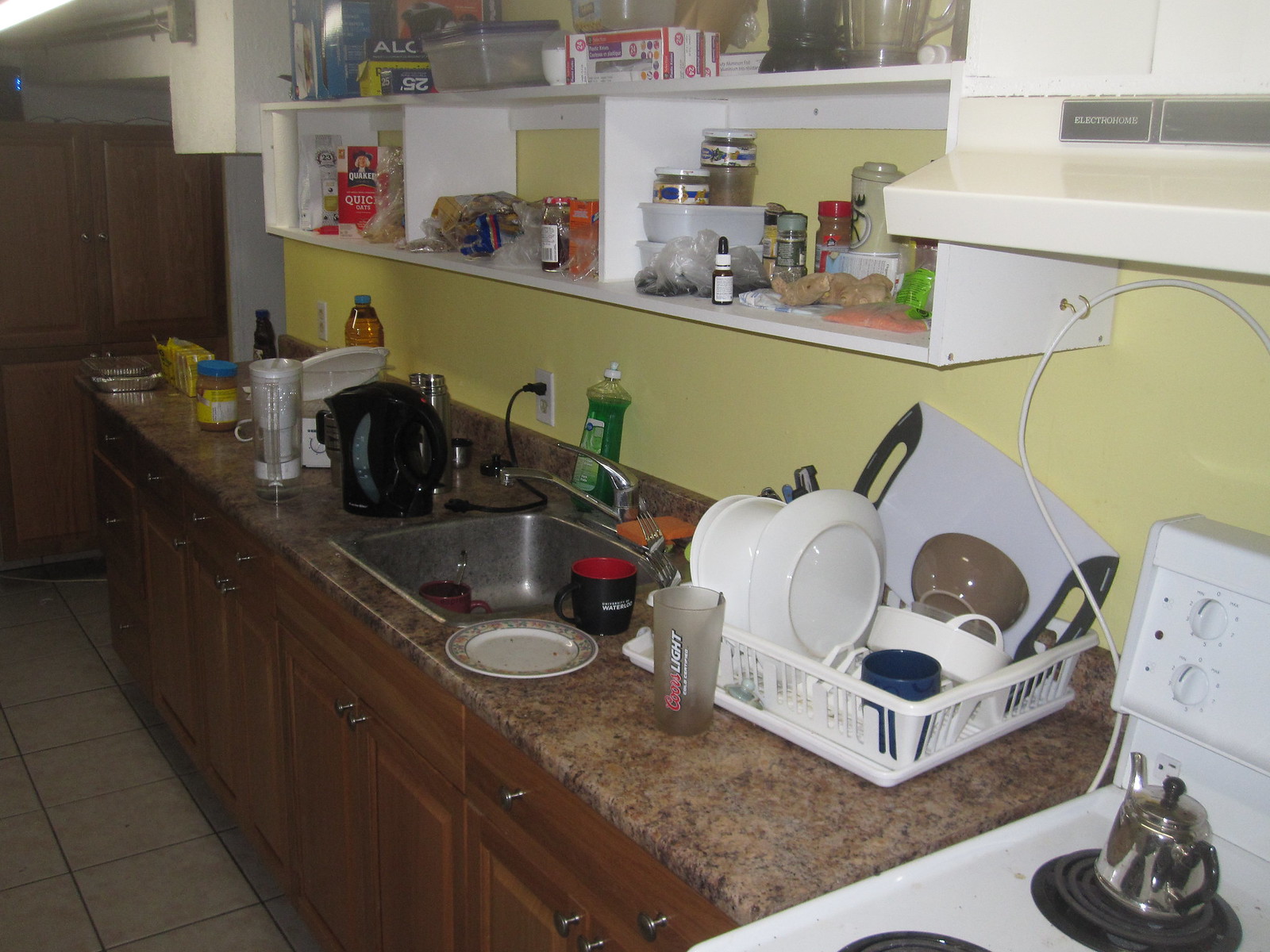This photograph captures a detailed view of a cozy, lived-in kitchen. On the lower right side, a white stovetop is prominently featured with a matching white hood above it. To the left of the stove, the brown and tan granite countertops gleam under the light, complemented by light brown cabinets beneath them. On the counter, a white dish dryer is neatly arranged with clean dishes, including a brown bowl, a dark blue cup, and several white plates. Next to the dish dryer stands a clear Coors Light glass.

Further down the counter, a sink comes into view with a red mug resting inside it. A black water boiler pitcher, which is plugged in, sits nearby, with green dish soap positioned behind the sink for easy access. Additionally, two white water pitchers accompany the black water pitcher, adding to the ensemble of kitchen essentials.

Toward the far end of the counter, a loaf of bread in yellow packaging and a jar of peanut butter with a yellow label and blue cap add a touch of color. Above the countertops are several white wooden shelves laden with various household items, including oatmeal, seasonings, assorted food articles, and Tupperware, all arranged to ensure convenience and functionality in this welcoming kitchen space.